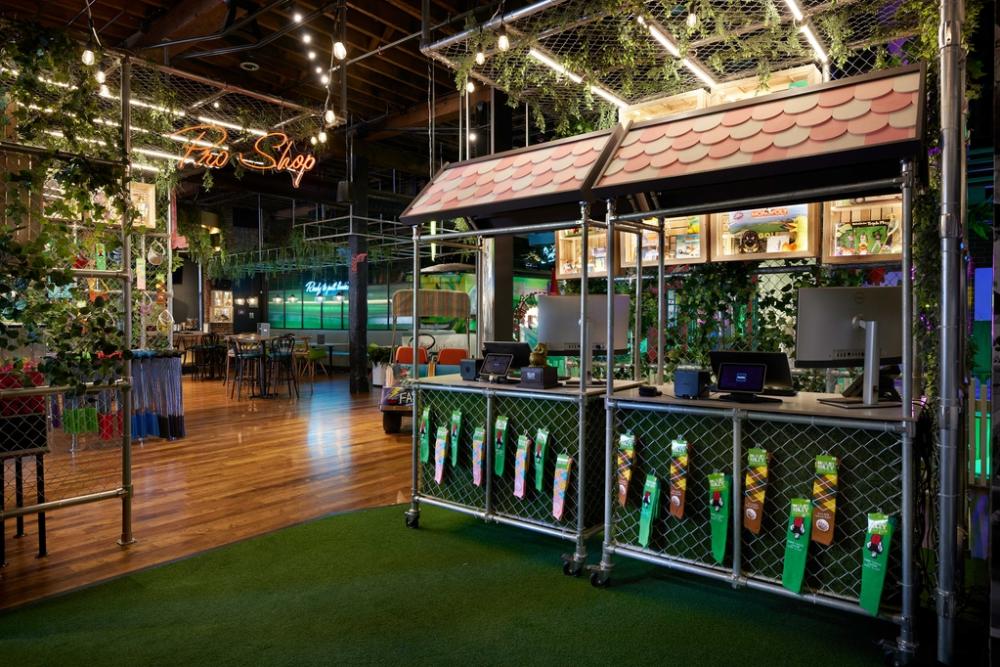The color photograph, taken in a landscape orientation and seemingly captured at night, depicts an indoor scene set in a convention center designed as a golfer's Pro Shop. Central to the image are two unmanned concession-like booths with monitors and cash registers, set against a dark green background adorned with golf-themed socks, some of which are mounted on a metal frame resembling a fence. The floor around these booths is covered with dark green artificial turf, while the rest of the area features a wood laminate floor. Suspended from the ceiling are strings of lights and numerous hanging plants, contributing to the elaborate atmosphere. To the left, tables and chairs are scattered in the background, suggesting additional shopping or lounging areas. Dominating the upper left corner, a neon sign glows in pink letters reading "Pro Shop." A golf cart, facing away from the camera, is parked on the right side of the image, enhancing the golfing theme. The environment is meticulously designed, blending realistic photographic elements to create an immersive Pro Shop experience for golfers.